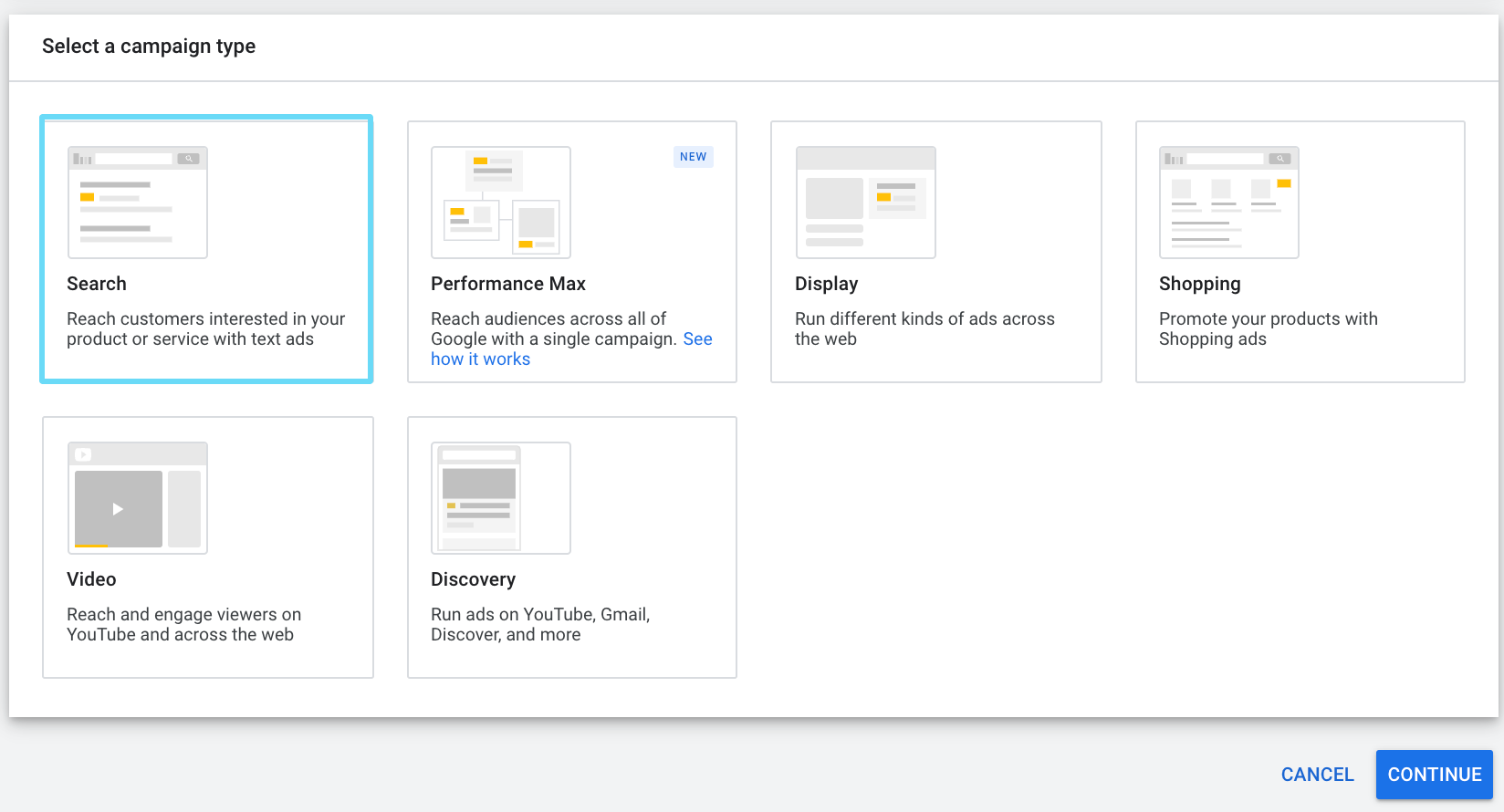This image is a screenshot from what appears to be an application or web design interface. The photo is rectangular, landscape-oriented, and approximately twice as long as it is tall, with a thin gray border that casts a subtle shadow, more prominent near the top and left edges. The background is primarily white. 

At the top, a thin horizontal gray line creates a border, and in bold black text, it reads "Select a Campaign Type." Below this, the interface is divided into two rows: the first row contains four boxes, and the second has two.

1. **Search Campaign**: The first box, slightly longer than it is tall, has a green border. It features an example webpage with gray and yellow lines and reads, "Search: Reach customers interested in your product or service with text ads."
   
2. **Performance Max Campaign**: The next box to the right has a label "New" in the top right corner. It states, "Performance Max: Reach audiences across all Google with a single campaign. See how it works."

3. **Display Campaign**: The third box reads, "Display: Run different kinds of ads across the web."

4. **Shopping Campaign**: The fourth box is labeled, "Shopping: Promote your products with shopping ads."

5. **Video Campaign**: The first box in the second row says, "Video: Reach and engage viewers on YouTube across the web."

6. **Discovery Campaign**: The final box reads, "Discovery: Run ads on YouTube, Gmail, Discover, and more." Each box also contains example webpage layouts with yellow lines, likely indicating where the ads will be displayed.

The provided screenshot effectively outlines various campaign options with descriptions and visual examples, helping users select the appropriate advertising strategy for their needs.